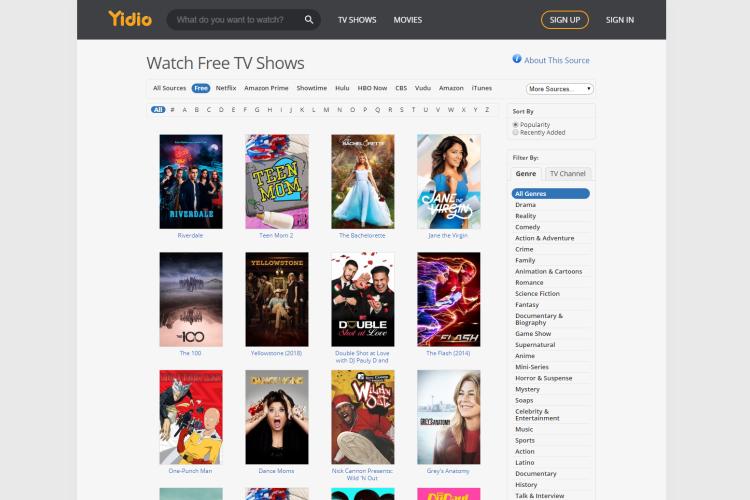The user interface (UI) of YIDIO features the brand name "YIDIO" prominently displayed in yellow text. Adjacent to this is a search bar containing the prompt "What do you want to watch" in faint lettering, accompanied by a white magnifying glass icon. The search bar is a dark gray, almost black, while the rectangle housing "YIDIO," the search bar, and the magnifying glass is a lighter gray.

Below, two main headings or menu paths for "TV Shows" and "Movies" appear in white text. On the far right side, there are "Sign Up" and "Sign In" buttons, with the "Sign Up" button highlighted by an orange oval. 

A section labeled "Watch Free TV Shows" is present, listing various streaming sources including Netflix, Amazon Prime, Showtime, Hulu, HBO Now, CBS, Vudu, Amazon, and iTunes, with an emphasis on free content. The options "Free" and "All" are highlighted by blue ovals, with "Free" currently selected.

Displayed in alphabetical order are all the letters from A to Z, followed by the 'not equal to' sign and a category labeled "All," which is also highlighted. The free TV shows listed include "Riverdale," "Teen Mom," "The Bachelorette," "Jane the Virgin," "The 100," "Yellowstone," "The Flash," "Double Shot at Love with DJ Pauly D" (partially cut off), "Dance Moms," "One Punch Man," "Nick Cannon Presents Wild 'N Out," and "Grey's Anatomy," all with corresponding icons. There are four more free shows partially visible but cut off.

To the right, an info icon with the label "About the Source" is visible, next to a drop-down menu labeled "More Sources." The UI offers sorting options by "Popularity" or "Recently Added," with "Popularity" selected by default. Filtering options are available by genre or TV channel, with the genre tab checked and "All Genres" focused. The genres listed include Drama, Reality, Comedy, Action and Adventure, Crime, Family, Animation and Cartoons, Romance, Science Fiction, Fantasy, Documentary and Biography, Game Shows, Supernatural, Anime, Miniseries, Horror and Suspense, Mystery, Soaps, Celebrity and Entertainment, Music, Sports, Action, Latino, Documentary, History, and Talk and Interview.